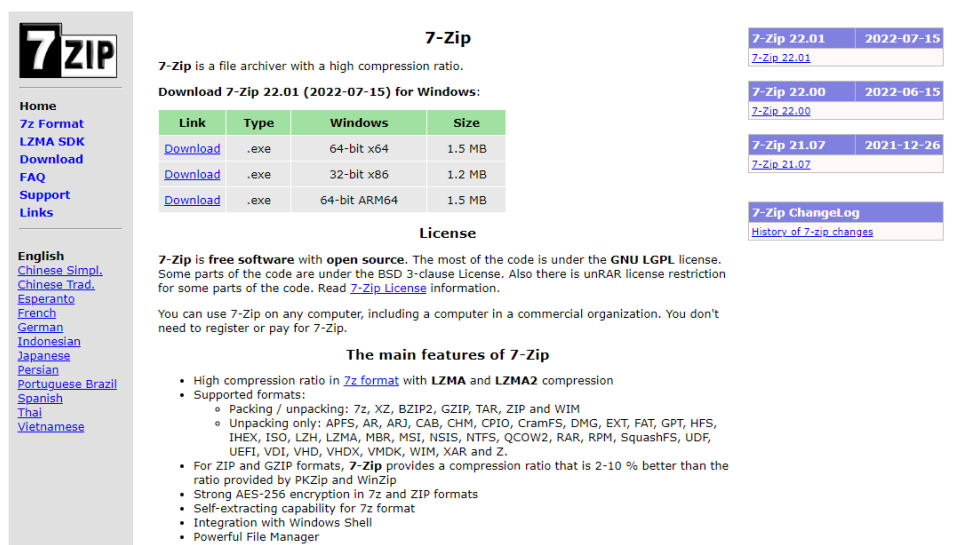Screenshot Description: 

The image is a screenshot of the homepage for 7-Zip, a file archiver software, presented within an interface that features a light gray background. On the left side, there is a vertical navigation menu topped with a prominent 7-Zip logo. Below the logo, the menu lists several items: "Home" in black text, followed by "7Z Format," "LZMA SDK," "Download," "FAQ," "Support," and "Links" all in blue text. Below these, another gray line separates the navigation items from the language options, starting with "English" in black, and followed by a list of about twelve different languages in blue text, ranging from Chinese to Vietnamese.

The central part of the screen, which occupies the majority of the space, has a white background. At the top, it displays the title "7-Zip" followed by a brief description, "7-Zip is a file archiver with a high compression ratio." Below the description, there is a download section featuring the text "Download 7-Zip 22.1-220715 for Windows." 

This section includes a table with a green header that categorizes the download options by "Link," "Type," "Windows," and "Size." The table contains three rows, each with a "Download" link. The "Type" column indicates that all links are in .exe format. The "Windows" column specifies the supported versions: 64-bit x64, 32-bit x86, and 64-bit ARM 64. The "Size" column lists the file sizes as 1.5 MB, 1.2 MB, and 1.5 MB, respectively. Licensing information is provided below the table.